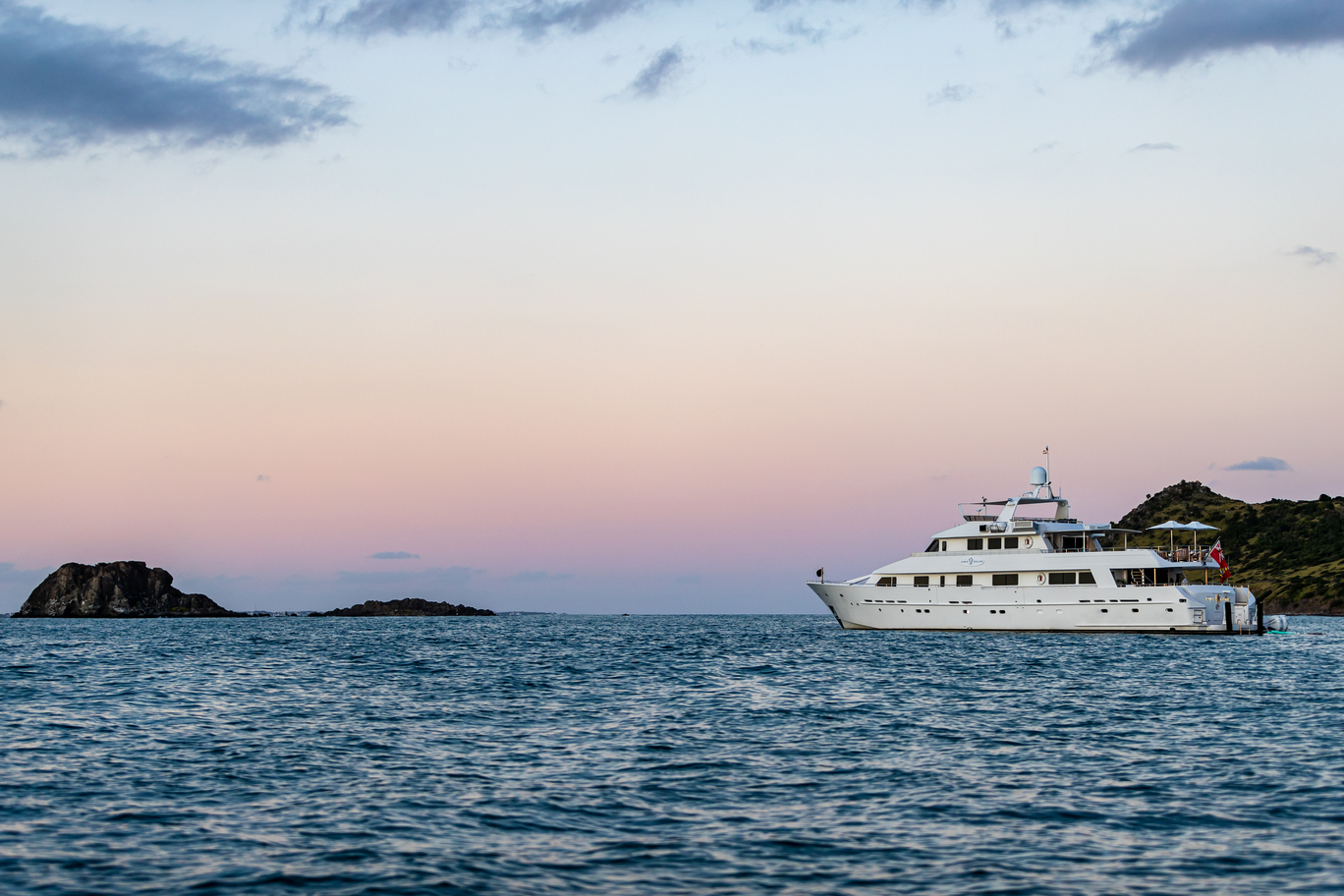The image captures a scenic moment at sea with a medium-sized white yacht gracefully navigating calm ocean waters toward the left. The yacht, featuring two and a half levels, is adorned with a small flag at the back and another at the top—one of which appears to be an American flag and the other a red flag of unknown origin. The upper deck boasts two umbrella-covered tables, and although no people are visible, one can assume there is at least a captain onboard.

In the background, a grassy, tree-covered hilltop is visible to the right, providing a lush contrast to the tranquil sea. To the left, rocky outcroppings and small, uninhabited islands add rugged beauty to the scene. The sky above transitions beautifully from pink and yellow hues near the horizon to a pale blue higher up, interspersed with darker, gray-blue clouds, indicating the approaching twilight. The serene ambiance and natural beauty make this a captivating and peaceful photograph.